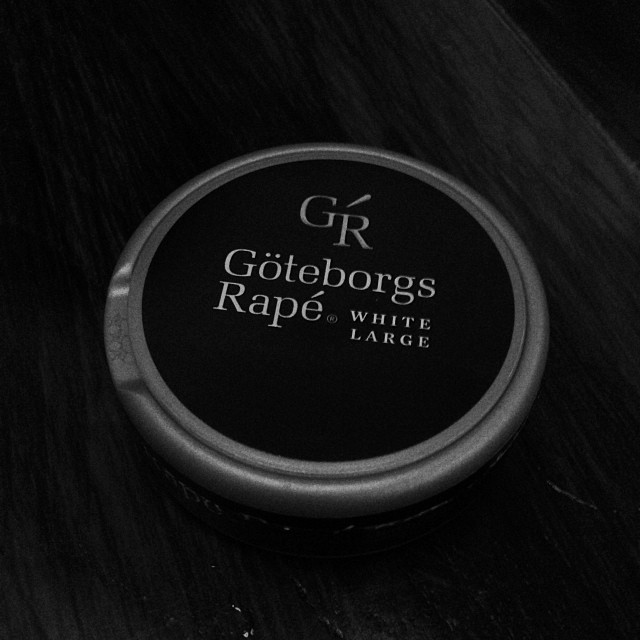The image depicts a small, circular canister, reminiscent of a compact or locket, made from gray or silver-toned plastic. It has a diameter of approximately one inch and features a slightly indented edge on one side, suggesting it can be opened. The top label, set within the canister's center, is black with white text. The prominent text includes "GR" with a decorative swoosh above the "R," followed by "Göteborgs Rapé," with an accent over the "é," and beneath that, "White Large." The canister is placed on a dark, black surface that appears to be either wood or fabric, although the exact material is indistinct due to the dim lighting and resolution. The black label on the top is the focal point, with a similar black label partially visible on the side. The overall atmosphere of the image is characterized by muted lighting and a close-up perspective.